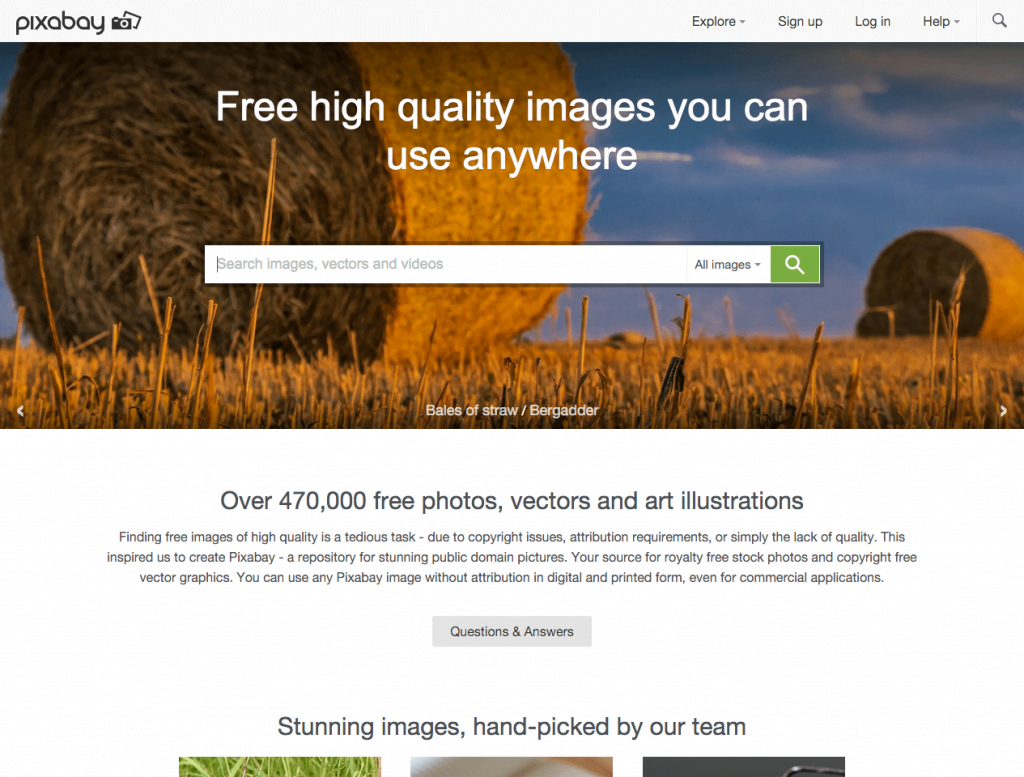This screenshot demonstrates the home page of the Pixabay website. At the very top of the page, there's a light gray horizontal bar. On the left-hand side, the word "Pixabay" is presented in bold black text next to an icon consisting of a black camera and a white image within it. On the right-hand side of the bar, several drop-down menus are visible with options labeled "Explore," "Sign Up," "Log In," and "Help," along with a search icon.

Beneath the gray bar, an image of a picturesque field with golden wheat and hay bales unfolds. Dominating the foreground is a single large hay bale, with another positioned farther back, both basked in a sunset ambiance under a bright blue sky with scattered wispy clouds. 

Overlaying this serene scene, white text proclaims, "Three high-quality images you can use anywhere." Directly below the image, a search bar invites users to find "images, vectors, and videos." To the right of the search field, a drop-down menu labelled "All Images" is available, followed by a prominent green search button.

Further down, descriptive black text states, "Bales of straw / Burr getter," followed by a concise summary touting the availability of over 470,000 free photos, vectors, and art illustrations. It explains the inspiration behind Pixabay: the challenge of finding free, high-quality images due to various copyright and attribution issues, and the site’s dedication to providing a comprehensive repository of public domain images. Notably, it highlights that images on Pixabay can be used without attribution in both digital and printed formats, even for commercial use.

At the bottom of the view, a gray box containing the text "Questions and Answers" invites users to engage further with the website's features and offerings.